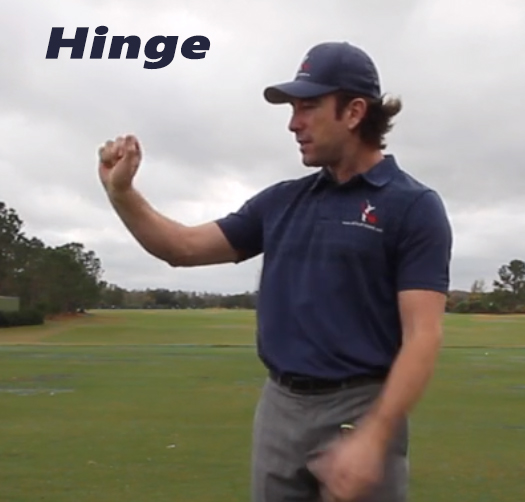The image shows a medium close-up of a man standing on a golf course under a cloudy sky. He's wearing a blue polo shirt with a small red and white logo on the left breast pocket, which matches the logo on his blue baseball cap. The man is engaged in a demonstration, gesturing with his right hand in a fist while his left hand is motion-blurred. He is dressed in gray pants and a black belt. The background features a low-cut green grass field typical of a golf course, with a few scattered trees. In the top left corner of the image, the text "HINGE" is prominently displayed in dark blue, suggesting a possible sponsor or event title. The man has brown hair that is visible from the back, and he is looking off to the left side of the frame.